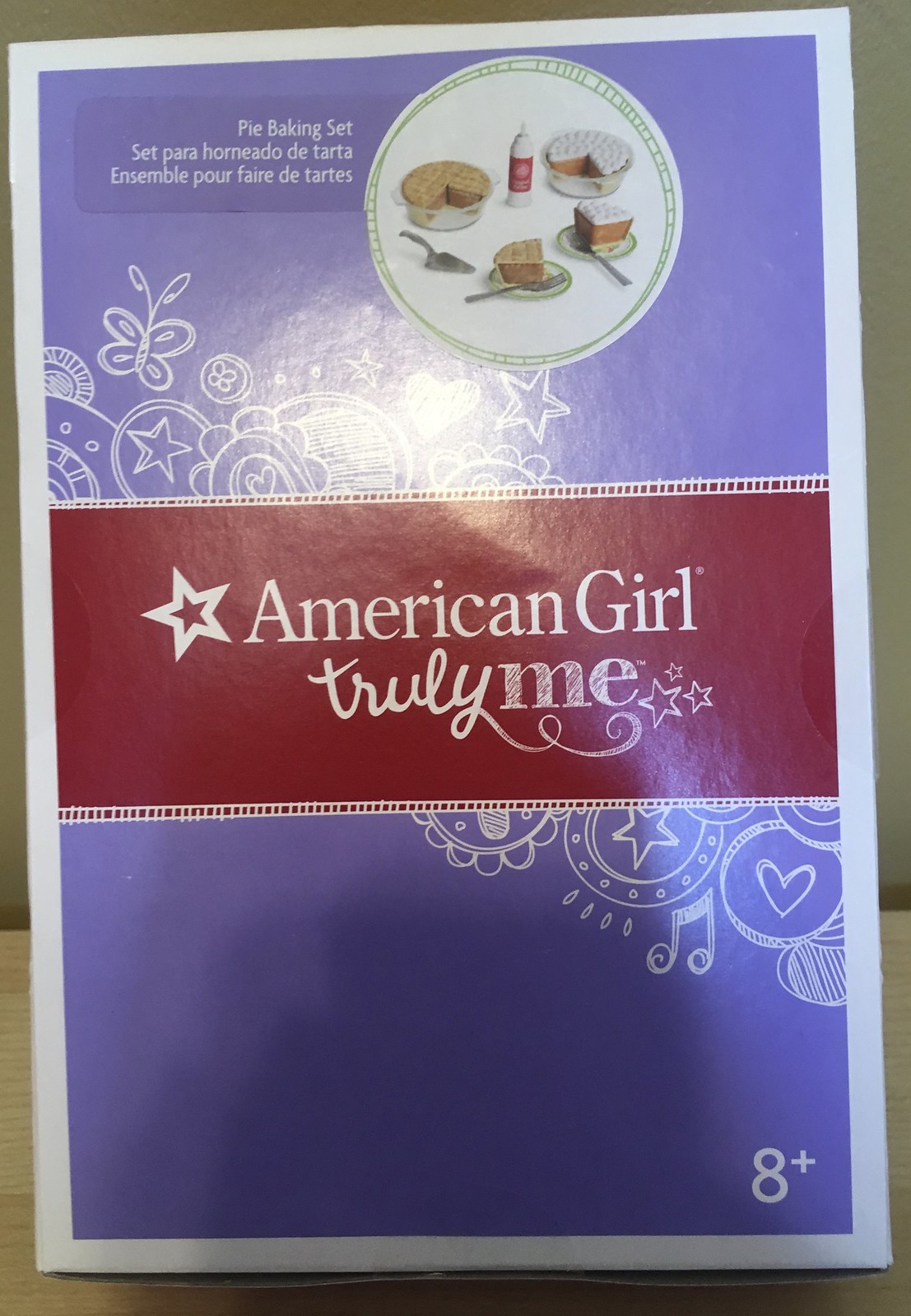The indoor color photograph captures a pamphlet cover with a bluish-purple background adorned with white sketches of butterflies, swirls, hearts, and music notes that flow diagonally across the design. The center of the pamphlet prominently features a red rectangular band with white text, which reads "American Girl" in bold letters accompanied by a cursive "Truly Me" with three stars to the right and an outlined star to the left of the "A" in "American." The upper portion of the pamphlet displays a white circle containing vibrant illustrations of a pie baking set, including two whole pies in clear pots, two wedges of pies on dishes, forks, a pie serving cutter, and a canister of whipped cream in the center. Adjacent to these images, the words "Pie Baking Set" appear. In the lower right corner of the pamphlet, the number "8+" indicates the targeted age group for this set, suggesting it is a toy baking set designed for children aged eight and up.